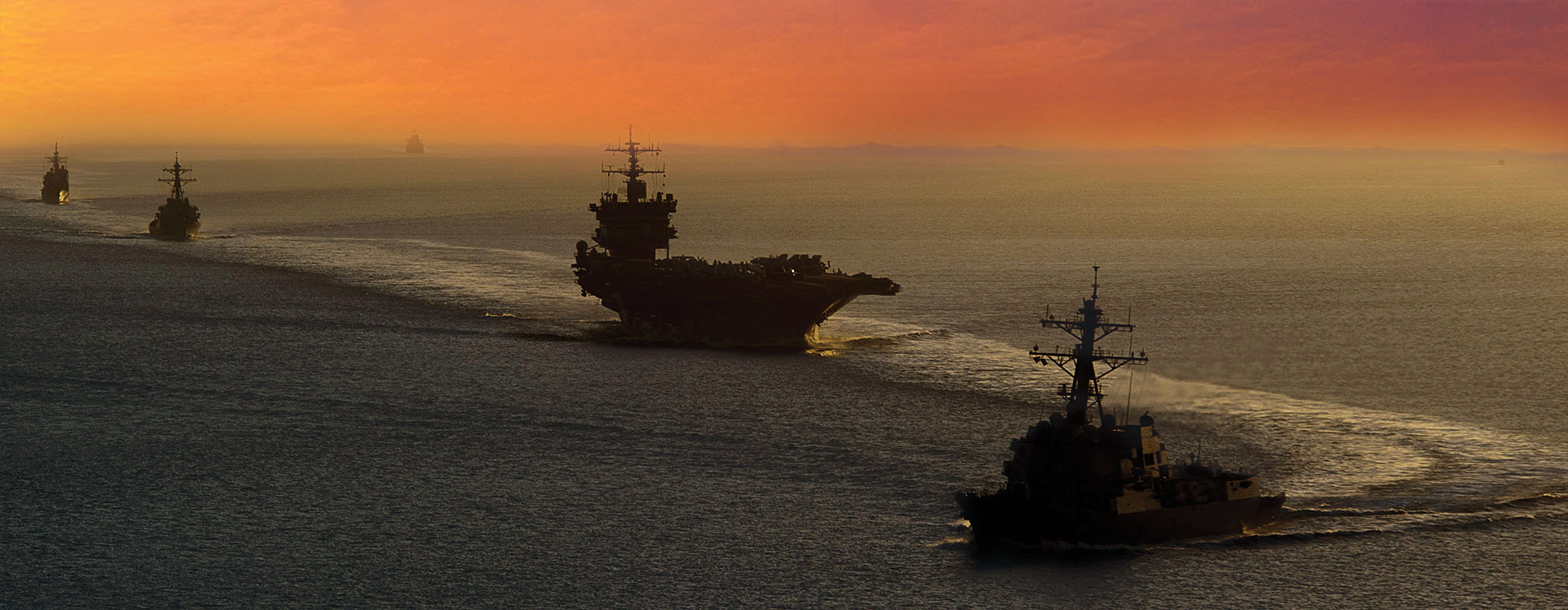In this evocative image taken during a low-light period, either at night, sunset, or sunrise, we see a serene yet striking scene of naval ships at sea. The water, a dull gray, reflects the fading light as the white wakes behind the ships create patterns on its surface. The sky is a captivating blend of orange and purple hues on the right, transitioning to lighter orange and yellow tones on the left. This gradient spectrum serves as a dramatic backdrop for the silhouettes of the ships.

We observe a formation of five large ships, characterized by their prominent antennas and equipment, indicating they are likely naval vessels. The arrangement is orderly: three ships are aligned in a row heading towards the horizon, one ship in the middle appears closer and more prominent, and another is situated in the lower right corner seemingly turning left to follow the others. Far in the distance, a very tiny ship can be seen on the horizon, adding depth to the scene. The calm water and the diminishing light emphasize the silhouettes, making the ships appear as dark shapes against the vibrant sky, creating a powerful and serene maritime landscape.